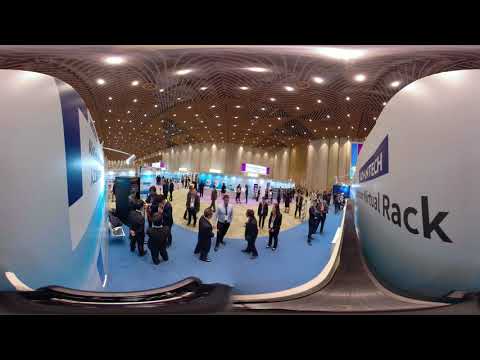This image shows the interior of a large convention hall filled with professional business attendees, many of whom are dressed in suits. The hall features a blue and cream-colored floor and a brown, ornately designed ceiling illuminated by multiple rows of circular white lights. The photograph has a curved appearance due to a fisheye lens, giving it a 360-degree view. The scene captures groups of people engaged in conversation, with several individuals standing near blue-colored stalls displaying various items, likely as part of a technology exposition. On the right side of the image, there's a banner with the word "tech" prominently displayed, and nearby, partially visible words like "tu-a-l" and "rack" hint at the technological theme of the event. The image is adorned with horizontal black strips at the top and bottom.